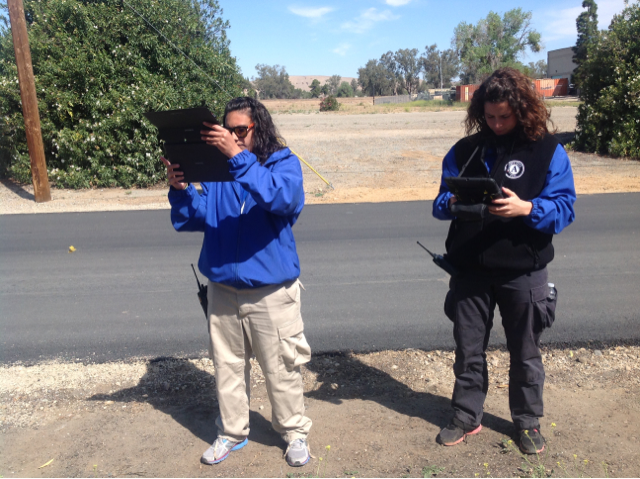In this outdoor scene, two individuals are standing beside a blacktop road, surrounded by a landscape of sparse trees and barren land. Behind them, nestled amidst the greenery, are flat-roofed buildings—one painted in red and another in gray. Both figures, a man and a woman, are dressed in utility-style clothing: cargo pants, casual shoes, and blue windbreaker jackets. Notably, the man wears a black vest adorned with a patch or emblem over a blue shirt, with his long hair flowing freely. The woman complements her beige cargo pants with a pair of light-colored sneakers and sports sunglasses over her long, dark hair.

Both are intensely focused on handheld devices that resemble tablets encased in rugged covers. Each carries a walkie-talkie device at their hip, the antennas visible, suggesting they are engaged in some sort of fieldwork or surveying activity. The man also appears to have a water bottle in one of his pockets. The somewhat rugged setting, with patches of dirt and stones near the road and a utility pole in sight, indicates a rural community or a remote area. The array of colors in the image includes shades of green, brown, blue, and red, contributing to the tranquil yet industrious atmosphere of this snapshot.